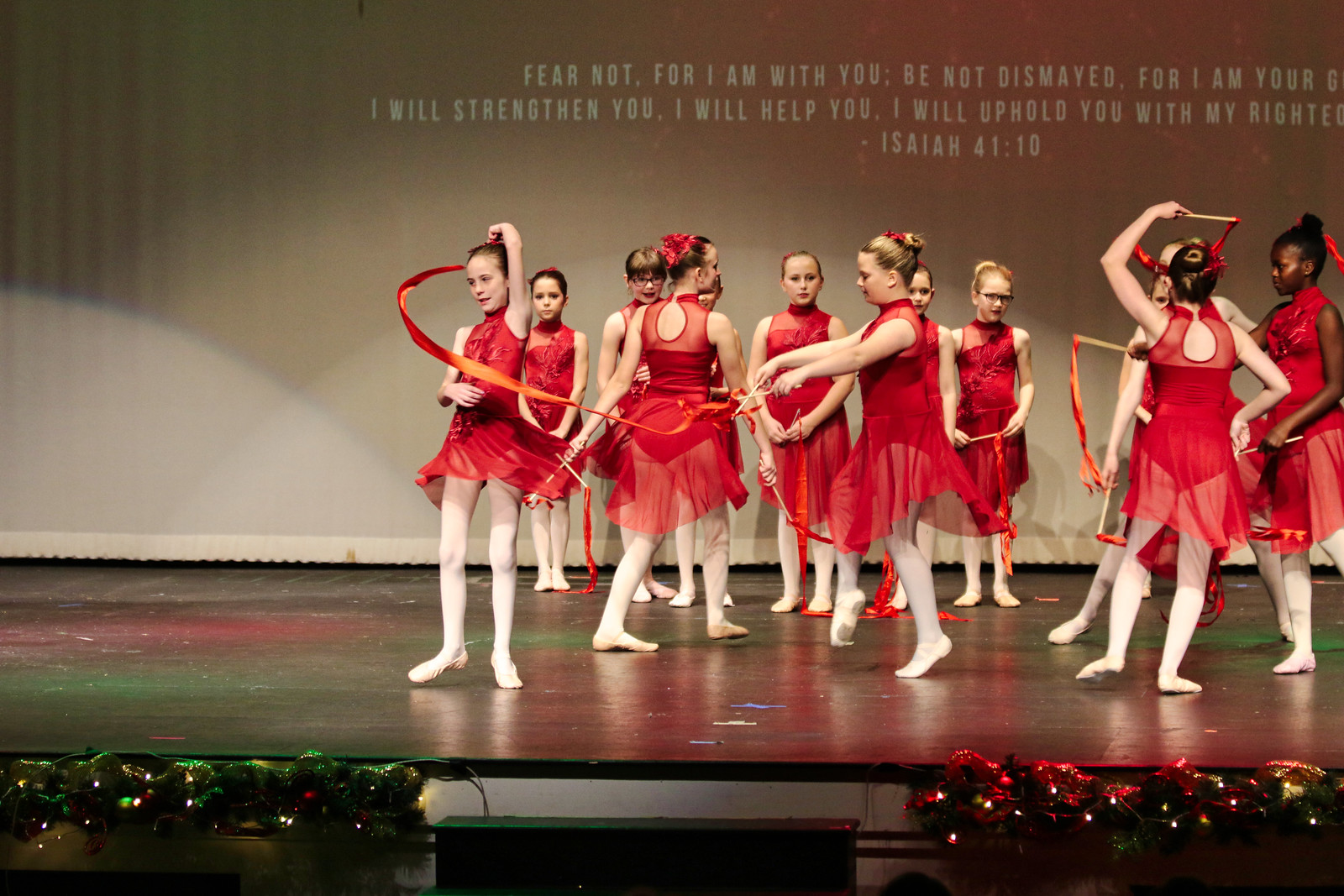The image shows a group of young girls, likely aged around 8 to 10, poised on a stage, dressed in coordinated red ballerina costumes accented with white tights and matching white ballet shoes. Each girl has her hair styled in a bun adorned with a red ribbon. Splashes of festive green and red stage lights highlight their forms against the black stage floor. Some of the ballerinas hold streamers on sticks, featuring golden-yellow hues. Framing the scene, Christmas lights sparkle along the edge of the stage, possibly indicating a holiday event. Behind the girls, a backdrop displays a passage from the Bible, Isaiah 41:10, in bold white capital letters: "Fear not, for I am with you; be not dismayed, for I am your God. I will strengthen you, I will help you, I will uphold you with my righteous right hand." Festive garlands with red and gold ribbons flank the stage, completing the warm, celebratory atmosphere.